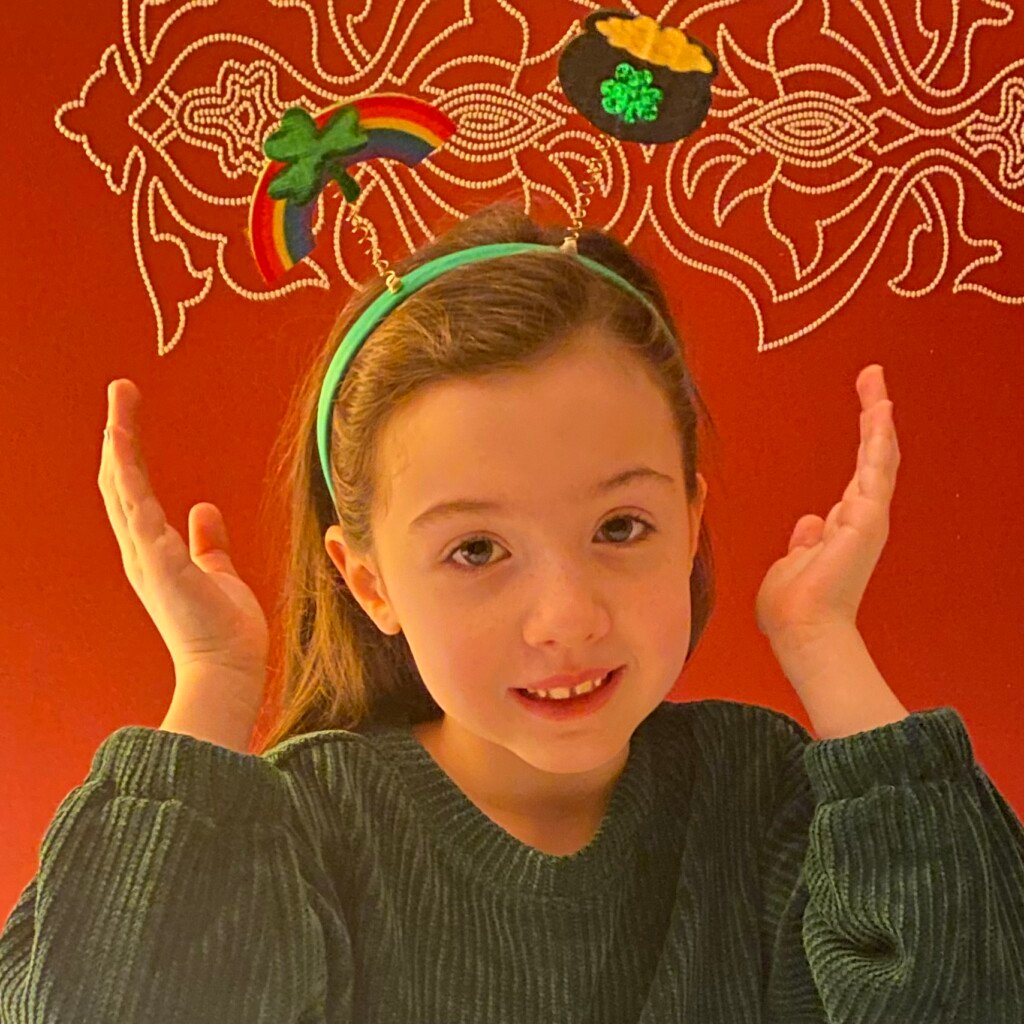This square photograph features a young Caucasian girl, approximately seven to eight years old, standing in front of a rust-colored wall adorned with abstract white beading near the top. The girl has long brown hair and big brown eyes that gaze directly at the camera, her face framed by a smile that reveals a gap between her front teeth. She's wearing a dark green corduroy long-sleeve shirt and a festive St. Patrick's Day headband. The headband has two playful coils sprouting from it: one side features a shamrock with a rainbow behind it, and the other side showcases a pot of gold with another shamrock. Her arms are raised beside her head, and she appears to be posing with a surprised or playful expression. A hint of lipstick adds a touch of color to her cheerful face.